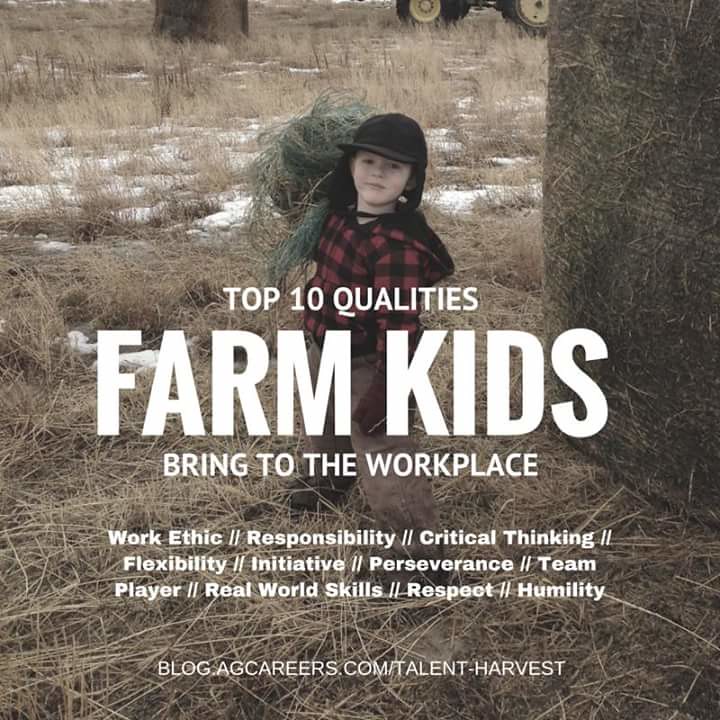The image is a color photograph combined with typography, resembling a poster designed to encourage bringing kids to work on a farm. Central to the image is a young boy, approximately six years old, dressed warmly for cold weather. He wears a red and black flannel-patterned parka with a hood, a dark hat with ear flaps, gloves, brown work pants, and possibly boots. The boy is carrying a bundle of hay over his right shoulder and stands amidst hay in front of a brick building, with snow covering parts of the ground. In the background, there's a tractor visible, adding to the farm setting.

Dominating the upper part of the image is white text that reads: "Top 10 qualities farm kids bring to the workplace." Below this headline, a list of qualities is presented in three lines, separated by slashes: "work ethic / responsibility / critical thinking / flexibility / initiative / perseverance / team player / real-world skills / respect / humility." The bottom of the image includes a URL: "blog.agcareers.com/talent-harvest," indicating the source of the advertisement, which highlights the benefits of involving children in farm work.